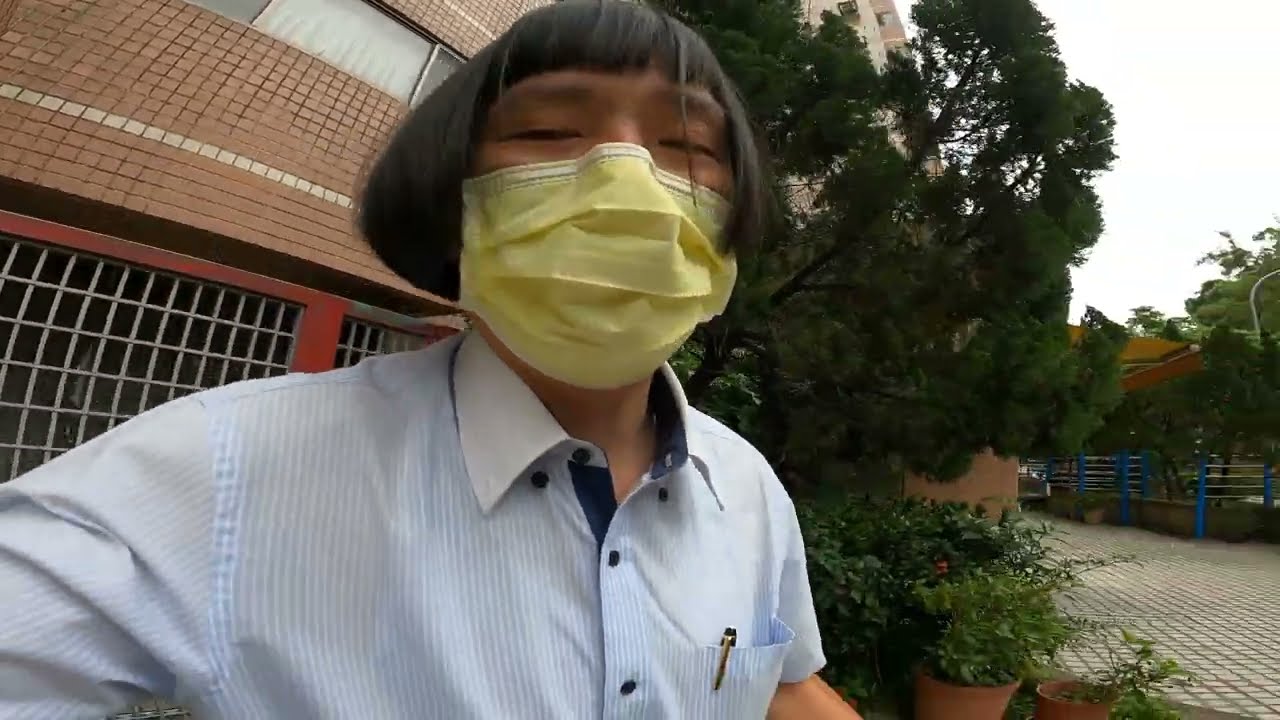The image is a poorly lit, full-color, outdoor selfie photograph taken on a cloudy day. The sky in the upper right is completely white, indicating thick cloud cover. The lush green trees and a fenced-in area with blue posts and bars are visible in the background. The subject, a young Asian individual with straight black hair in a pageboy haircut, is wearing a yellow mask that covers most of their face and a short-sleeve blue pinstriped button-up shirt with a collar. A black pen is tucked into the chest pocket of the shirt. On the far left, there's a beige brick or stone building with a red-framed door, adorned with a silver small grid work, and windows overhead. To the right of the individual, a gray cobblestone path is bordered by trees and potted plants. The setting appears to be an urban or apartment complex area devoid of cars, suggesting the subject is either out for a walk or engaged in some daily activity within the residential complex.